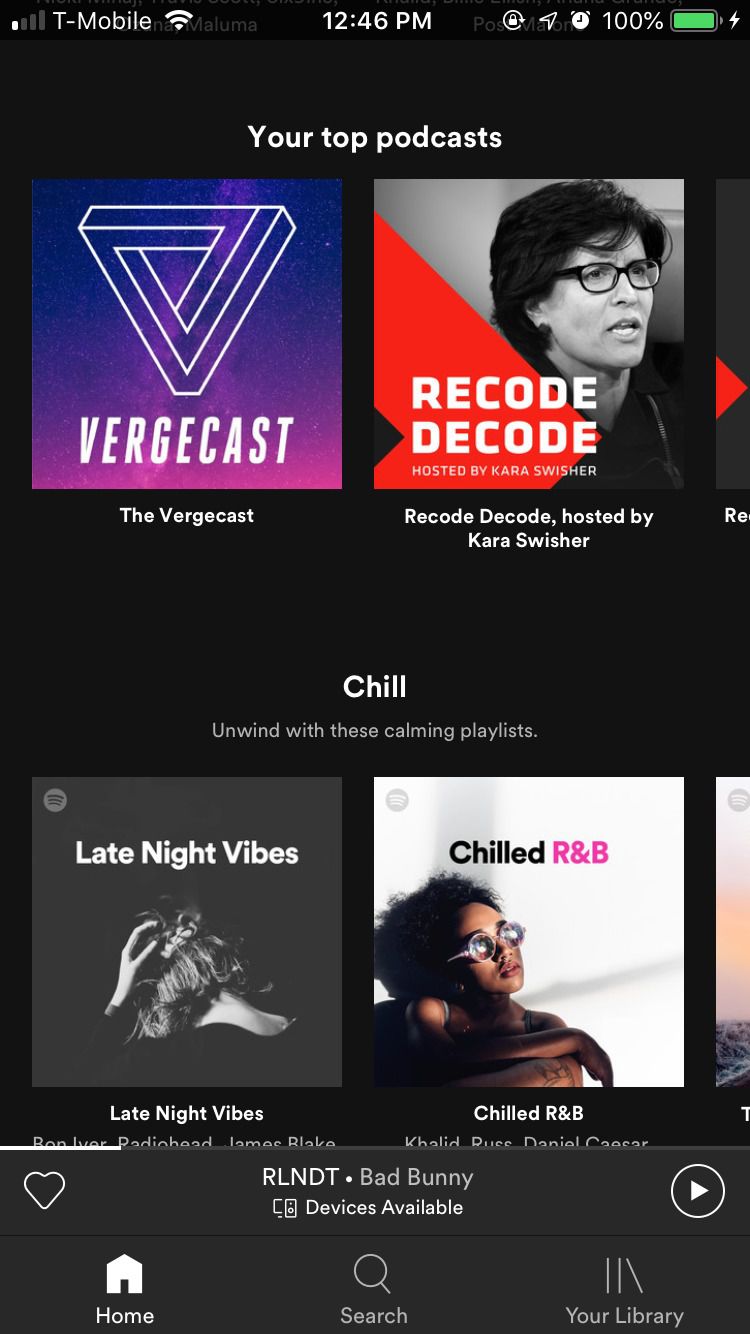The image showcases a cell phone screen displaying a music platform interface. At the top left corner, the status bar indicates "T-Mobile" next to a Wi-Fi icon. The time is displayed in the center as 12:46 PM, while the top right corner shows three additional icons and a fully charged battery at 100%.

Below the status bar, the header "Your Top Podcasts" is prominently displayed. Under this header, two podcast thumbnails are featured side by side. On the left, the podcast titled "The Vergecast" is presented with an image characterized by a predominantly purple background transitioning to pink at the bottom. The logo features a white-outlined triangle with the word "Vergecast" beneath it in white text.

To the right, the podcast "Recode Decode" hosted by Kara Swisher is highlighted. The image includes a black-and-white portrait of Kara Swisher, identifiable by her glasses and short black hair. The left side of the image is bright red, with the podcast title "Recode Decode" written in white text.

Below the podcasts, there is a playlist titled "Chill." Within this playlist, two tracks are shown. On the left is "Late Night Vibes" and on the right is "Chilled R&B," which has a white background featuring a person with glasses and a dark brown shirt.

Currently, the song "RLNDT" by Bad Bunny is in progress, with a heart icon to the left for favoriting and a play icon to the right for playback control.

At the bottom of the screen, there are three navigation icons against a black background: "Home" on the left, "Search" in the middle, and "Your Library" on the right.